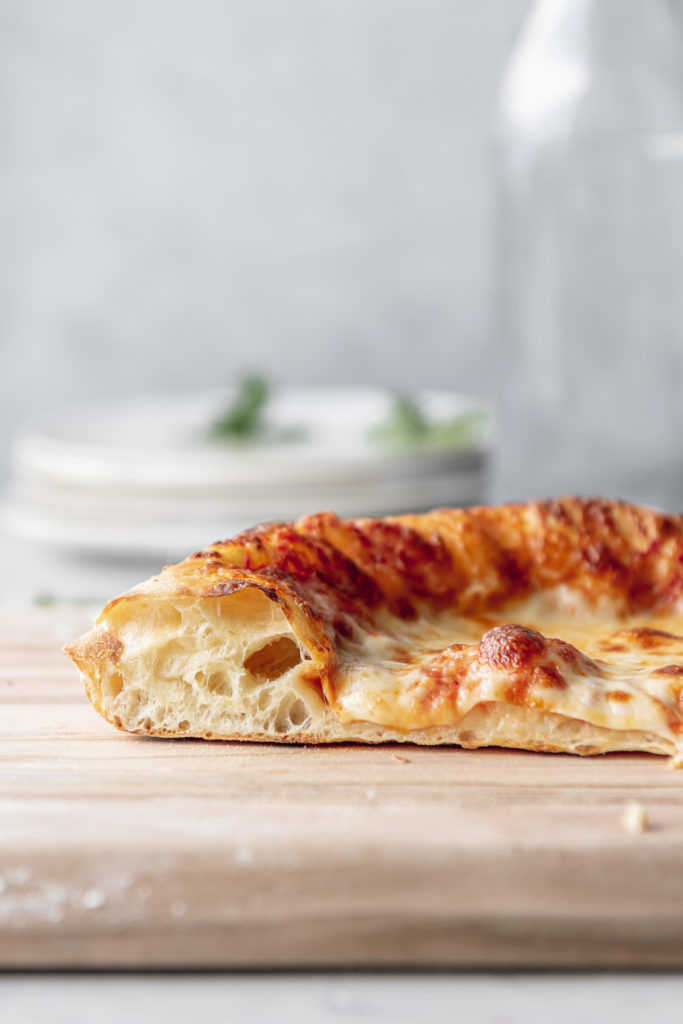The image features a close-up shot of a slice of cheese pizza placed on a brown wooden cutting board. The focus is mainly on the pizza, revealing its slightly crisp, darkened crust, and doughy interior. A portion of the melted cheese is visible, though no other toppings can be identified. Surrounding the pizza are small crumbs scattered on the board. The pizza appears to be quite thin, likely homemade. In the blurred background, one can discern a white kitchen setting with a white countertop, a pot with green leaves, plates with bits of food, and a bottle, possibly made of glass or plastic. The overall scene suggests a casual, everyday kitchen environment.